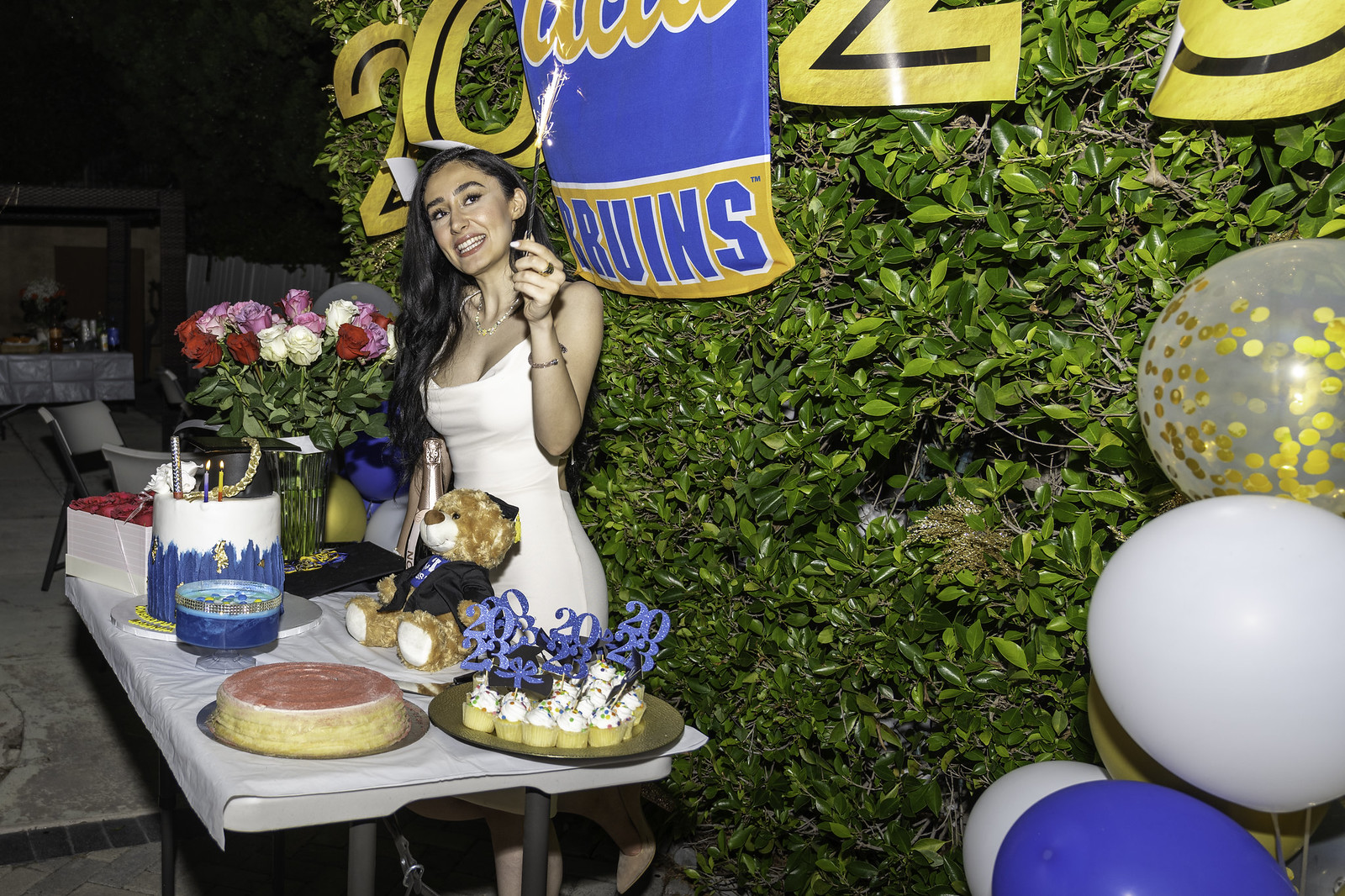In this vibrant, nighttime photograph, a young lady stands behind a festive table adorned with a white tablecloth, amidst a celebratory setting likely related to UCLA Bruins in 2023. Dressed in a sleeveless, white dress, the lady, with shoulder-length dark hair, smiles warmly into the camera, her left hand holding a wand-like firecracker. A black necklace graces her neck, with a bracelet and ring adorning her left hand's middle finger. Behind her, tall greenery appears, decorated with the numbers "20" and "23" in yellow, although the top of the frame cuts off the second "20," and a blue banner that reads "UCLA Bruins."

The table in front of her features an array of food items and decorative touches. A tall cake with white and blue icing and two candles holds center stage, accompanied by a smaller pink-frosted cake, cupcakes topped with "2023" decorations, a tray of assorted pastries, and a couple of pies. Beside these treats is a bouquet of red, white, and pink roses in a vase and a golden teddy bear wearing a dark vest, leaning against the lady. Gifts and a champagne bottle also add to the celebratory ambiance. The right-hand side of the photo reveals a bunch of balloons—blue, white, and one translucent with gold flecks. Wooden fences and a night sky form the backdrop of this joyous occasion, suggesting an outdoor celebration.